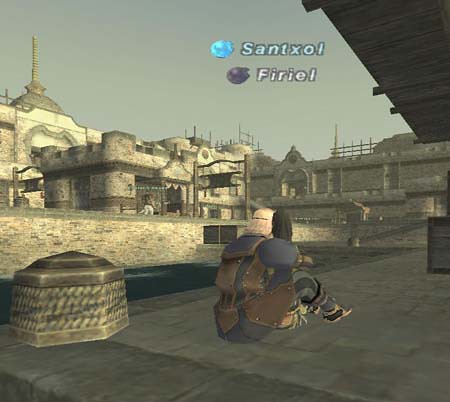The image is a screenshot from a video game depicting a large, stone porch area with a well encased in a cylindrical stone structure in the background. In the foreground, an older man with blondish or white hair is seated on the ground, holding a child on his lap. He is wearing a puffy blue shirt or jacket with brown leather-like sections and possibly a backpack. His knees are bent and his feet are flat on the cobblestone ground. To the upper left of the structure, a castle or large stone building is visible, with a person in white moving around inside. At the top of the image, there are two roundish icons with fireball-like appearances: a light blue one labeled "SANTXOL" and a darker purple-black one labeled "FIRIEL". The scene is dominated by a brown and gray color palette, under a gray sky. The graphical style suggests it might be from an older console game, such as PS2, Xbox, or PS3.